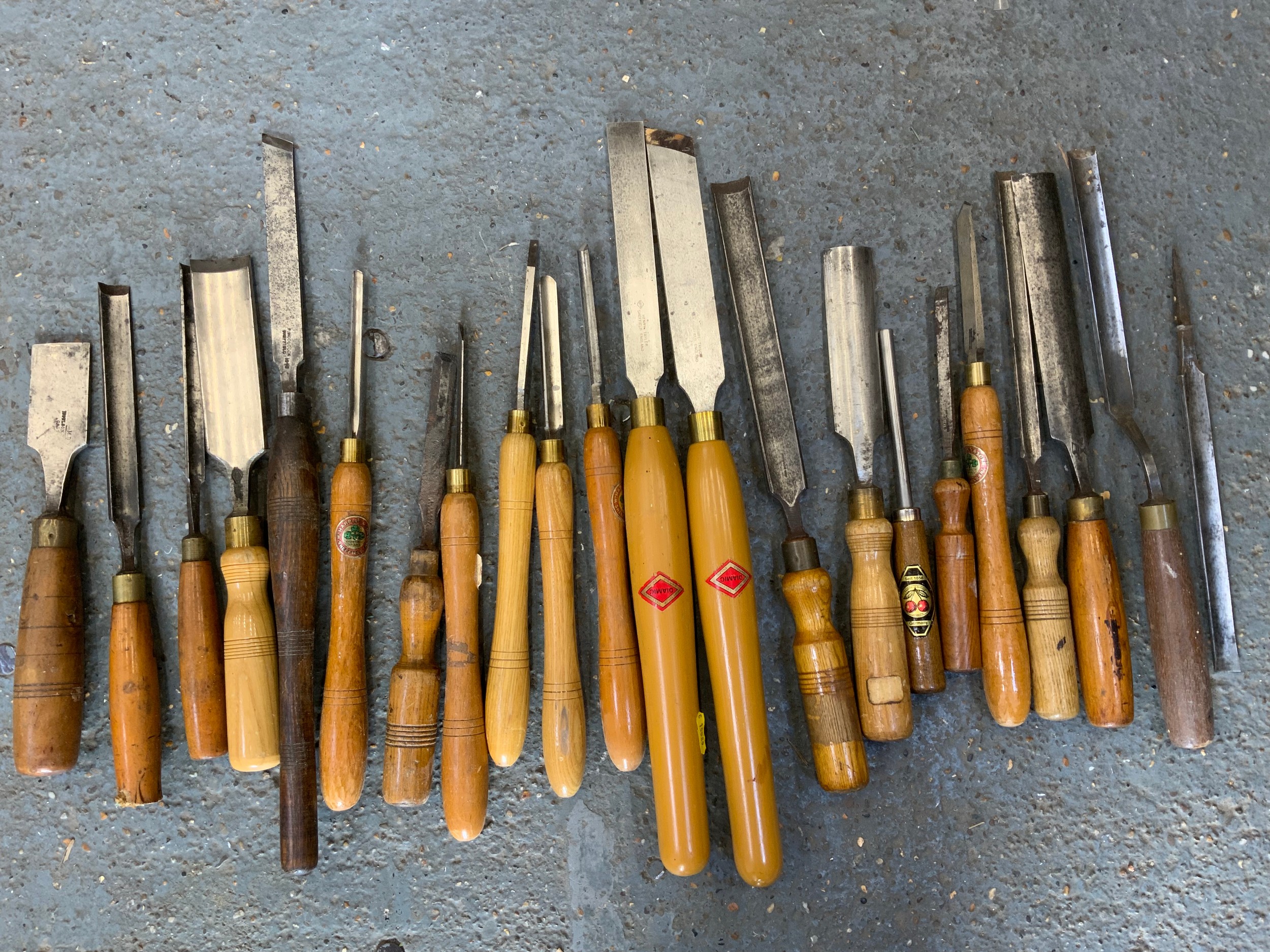The image displays an assortment of woodworking files meticulously arranged on a gray, concrete-like or bluish asphalt surface that covers the entire frame. Each file is laid out horizontally, with their wooden handles at the bottom and the metallic filing surfaces pointing upwards. These tools vary significantly in size and shape, with some resembling knives and screwdrivers, featuring wide to narrow and long to short profiles. The wooden handles exhibit a range of hues, from dark to light brown, and some even have distinct designs. Notably, one file on the far right lacks a handle and is purely metal. The arrangement is such that, although there is no specific pattern, the handles are uniformly placed at the bottom, creating a visually appealing display of tools ready for use.